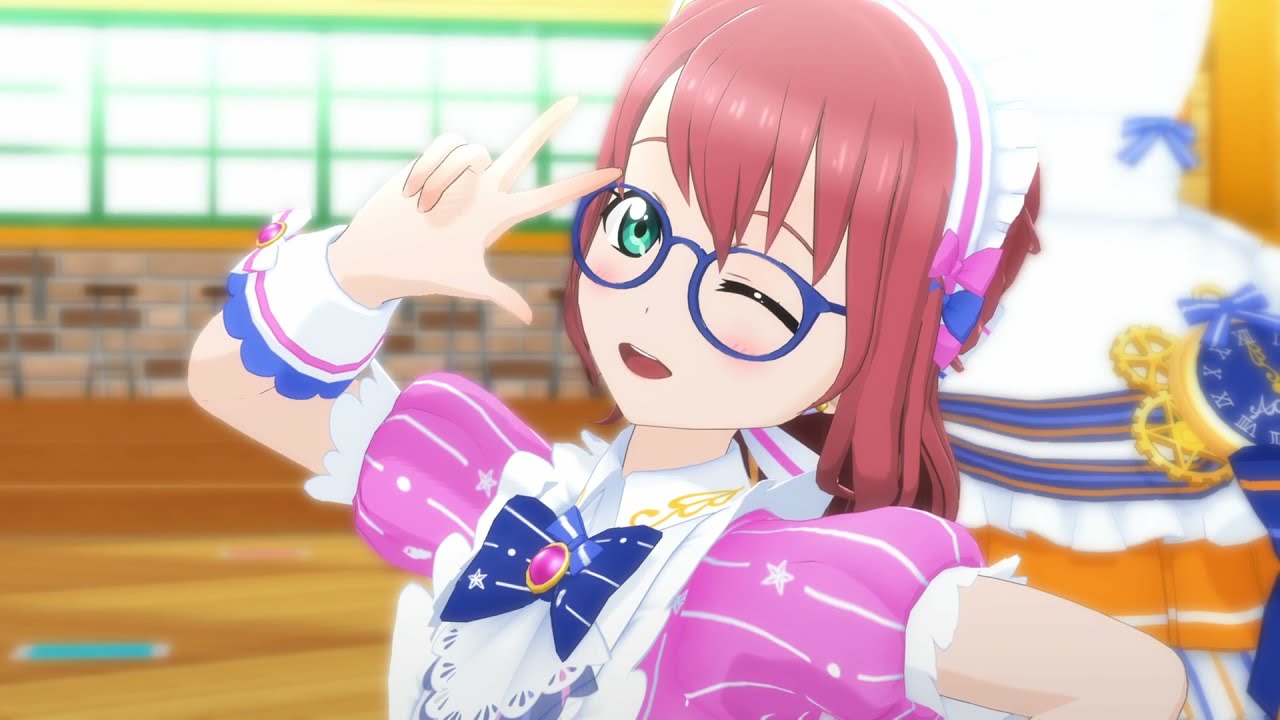The image depicts an anime girl in a school gym setting, standing in front of a tan and dark brown brick wall. Above the wall, there's a rectangular section composed entirely of windows with green frames. The girl is centrally positioned and appears to be posing for a picture, reminiscent of a camera mode in a video game. She wears a pink blouse with puffy short sleeves that extend to her upper arms and a white chest area, adorned with a blue bow tie featuring white stripes, stars, and dots. A purple pendant with a gold ring accentuates the bow. Her outfit includes a white apron-like front and a trim detailed with frills and intersecting white stripes, stars, and dots. She has long, red hair that flows down her back, and she tilts her head to the right while winking with her left eye. Her right eye, which is open, reveals a green iris beneath blue-rimmed glasses. A pink and white headband with small bows complements her look. She holds her left hand up near her face, gesturing a peace sign with her thumb, pointer, and middle fingers extended. In the background, the gym room appears somewhat blurred, possibly with another dress visible off to her right.